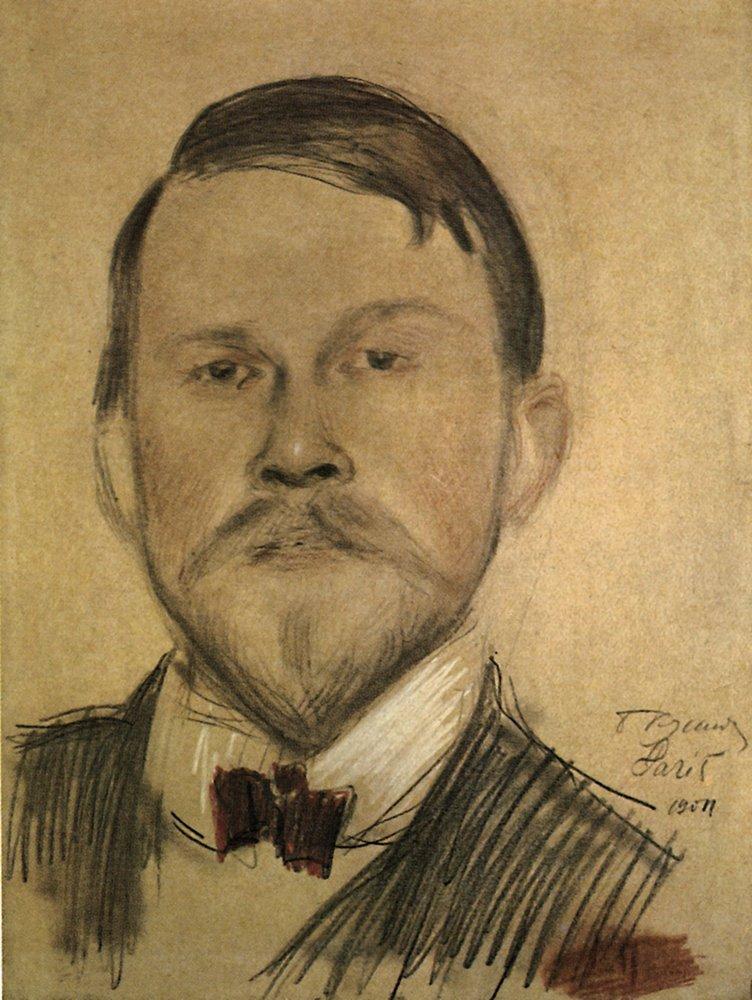The image portrays a detailed sketch of a man drawn on yellowish parchment-like paper with gray shading throughout. The man is depicted from the upper chest up, gazing directly outward. His short, dark hair is swept to the right, and he sports a goatee and a thin mustache, giving his chin a distinct pointy appearance. His attire consists of a formal black suit, a white shirt, and a red bowtie. Highlights are especially noticeable on his nose and cheeks, the latter having a slight pinkish shade. To the right of his jacket, a partially legible signature includes the word "Paris" and the year "1904," with a red brushstroke marking the bottom of the sketch.